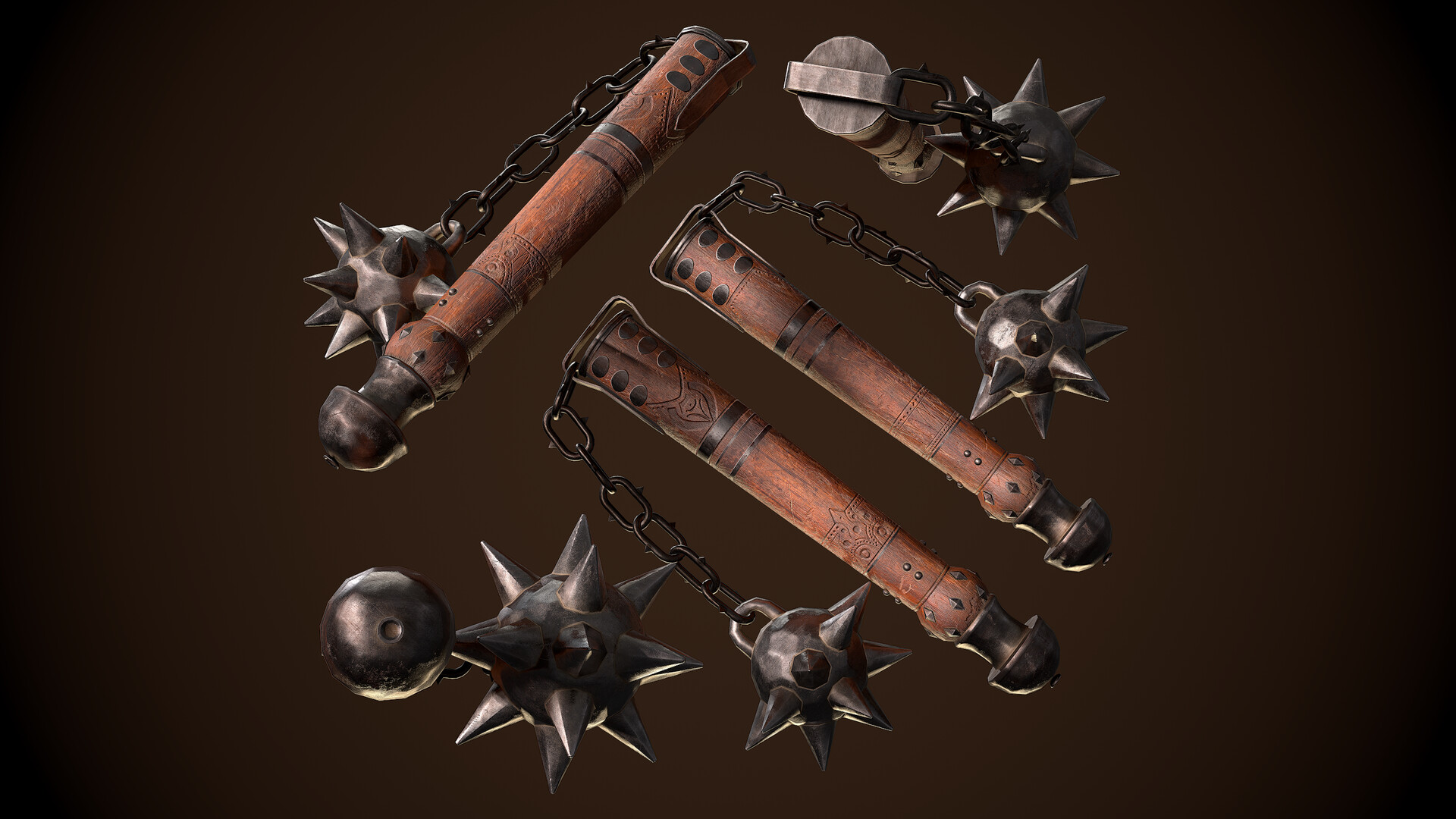The image depicts a digital rendering of a medieval weapon known as a morning star, set against a gradient background that transitions from dark black to lighter brown at the center. The weapon features long, thin wooden handles, tinged with reddish-brown, and iron bands encircling them. Attached to the end of the handles by approximately a foot of chain is a spherical, metallic ball spiked with large, black points. This menacing object is presented multiple times within the image, showcasing varied perspectives from above, below, and the sides, which appears to be an asset intended for use in a 3D digital environment, such as a video game or animation. Overall, it's a highly detailed and vividly rendered demonstration of this destructive medieval tool.